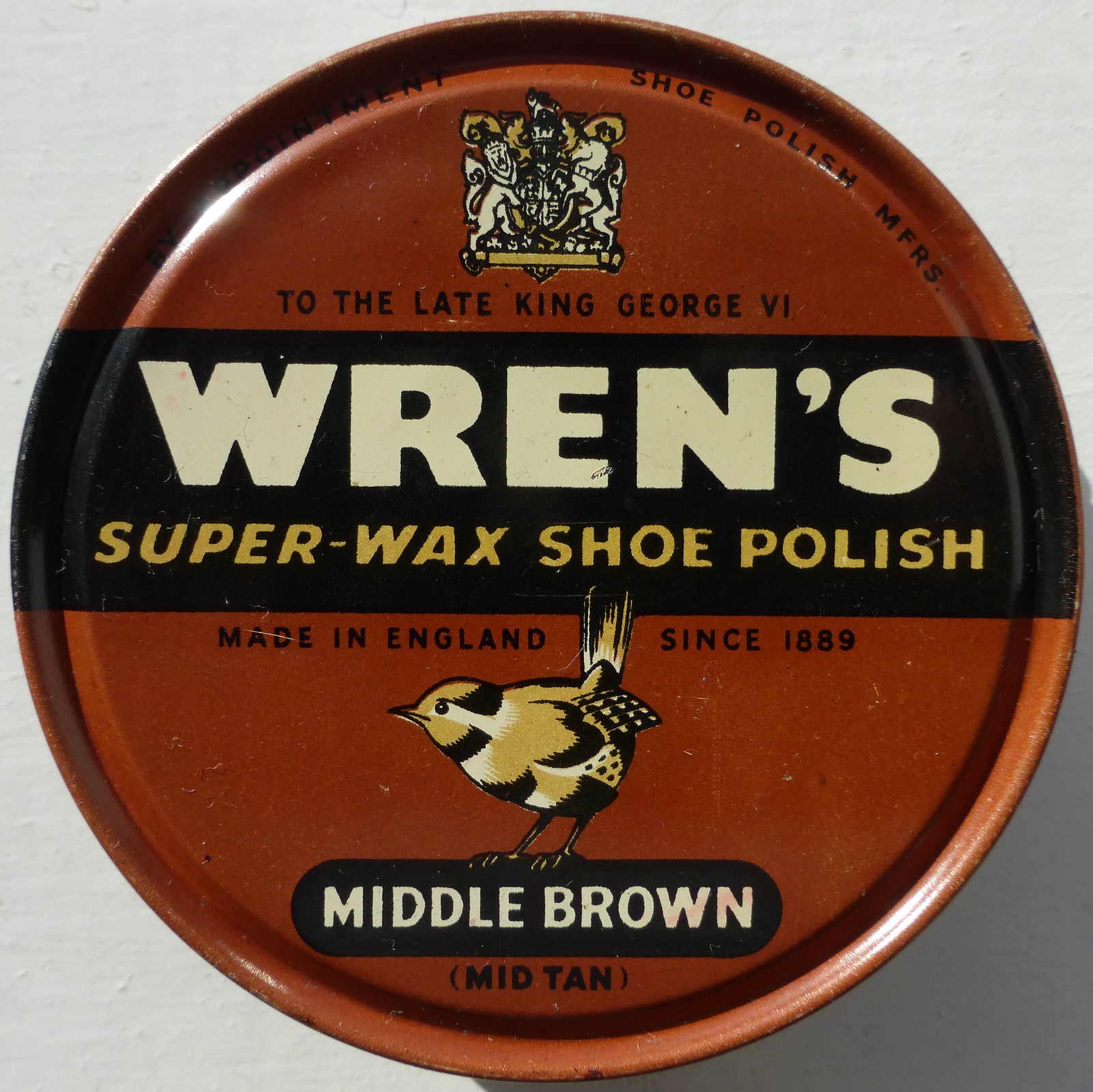The detailed image depicts a circular lid of a tin, prominently placed in the center and occupying almost the entire rectangular frame with a light grey background. The lower right corner is shadowed, creating a darker grey hue. The tin's lid is primarily brown with detailed engravings. At the top, there's a historic gold and white crest featuring a lion on the left and a unicorn on the right, flanking a central tower. Just below this crest, black text reads: "By appointment to the late King George VI."

A distinct black horizontal banner across the center of the lid prominently displays "Wren's Super Wax Shoe Polish" in large white letters. Supplementing this, small black text below the banner states, "Made in England since 1889". At the bottom of the lid, a carefully illustrated wren in gold and black stands in front of an oval-shaped black background. Inside this oval, white text announces the color, "Middle Brown," with "Mid Tan" in parentheses below. The overall style and layout suggest this image could be used for marketing on a website selling shoes or shoe polish products.